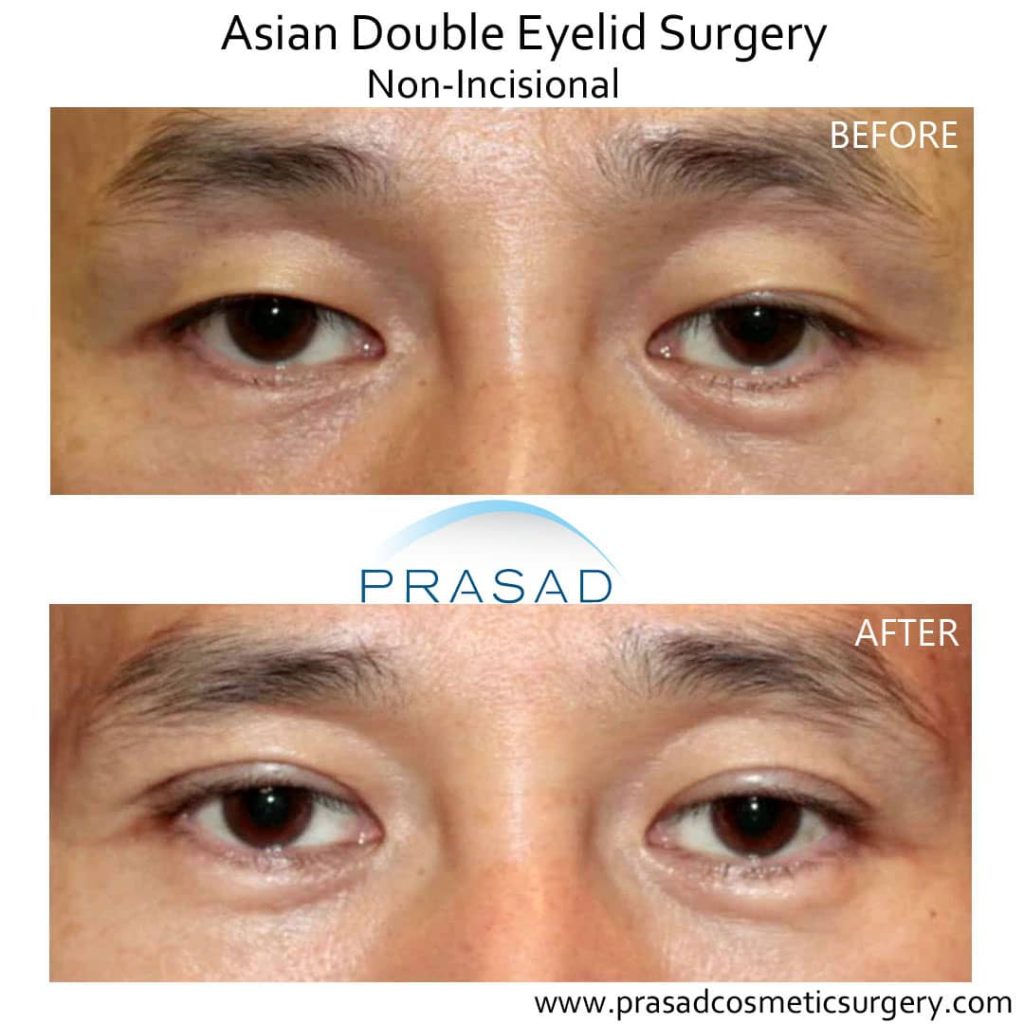The image features two color photographs, showing a close-up view of an Asian man's eyes, before and after a non-incisional Asian double eyelid surgery. The top of the image is labeled "Asian Double Eyelid Surgery, Non-Incisional" in black text against a white background. Below this, the "before" photograph shows the man's eyes without a noticeable fold in the eyelids. In the middle of the image, there is a blue logo with the word "PRASAD" beneath a blue rainbow arc. The "after" photograph at the bottom shows the man's eyes with a newly created fold, indicating the results of the surgery. Along the bottom edge, the website "www.prasadcosmeticsurgery.com" is displayed in black text.